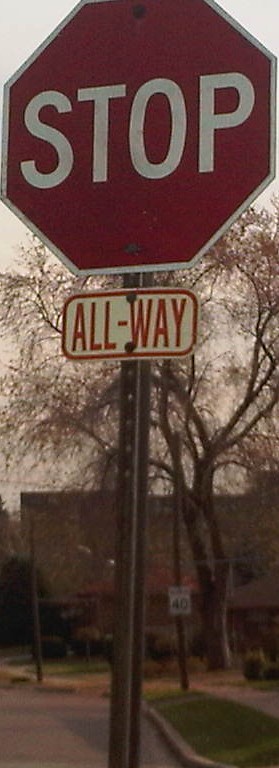This photograph captures a stop sign at a corner in a residential neighborhood on a gray, cloudy day. The stop sign, slightly cut off at the top and filling the narrow, vertical frame, is the classic red octagon outlined in white with bold white letters spelling out "STOP." Below it, a smaller rectangular sign with red writing on a white background reads "ALL WAY," indicating that all four corners of the intersection are stops. In the background, there's a brick building that's a bit blurry, with a red structure that could be an umbrella or a roof. The scenery reveals it's late fall; the nearly leafless trees add to the somber atmosphere. A nearby street sign indicates a speed limit of 40 miles per hour. Overall, the image has a vintage feel, reminiscent of photographs from the 60s or 70s.